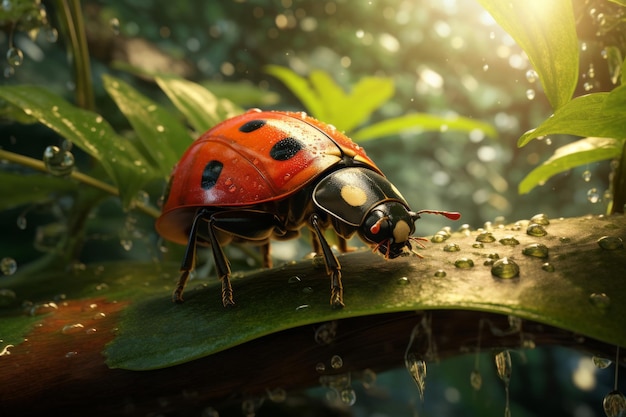In this highly detailed and close-up photograph, a vibrant ladybug stands prominently on a leaf adorned with glistening dew droplets. The ladybug's striking red shell is decorated with distinct black spots, and its black head features yellow markings along with delicate antennae. Fine fur-like structures and the intricate details of its legs are clearly visible as they grasp the leaf. Surrounding the ladybug, the leaf and its surface display beautifully formed water droplets, reflecting the scene’s recent rain. The background, though blurred, conveys a lush greenery with more dew-coated leaves, suggesting a verdant and sunny environment highlighted by glimmers of sunlight filtering through. This image captures the delicate balance between the natural world and the intricate beauty of the ladybug amidst its vibrant, dewy green surroundings.